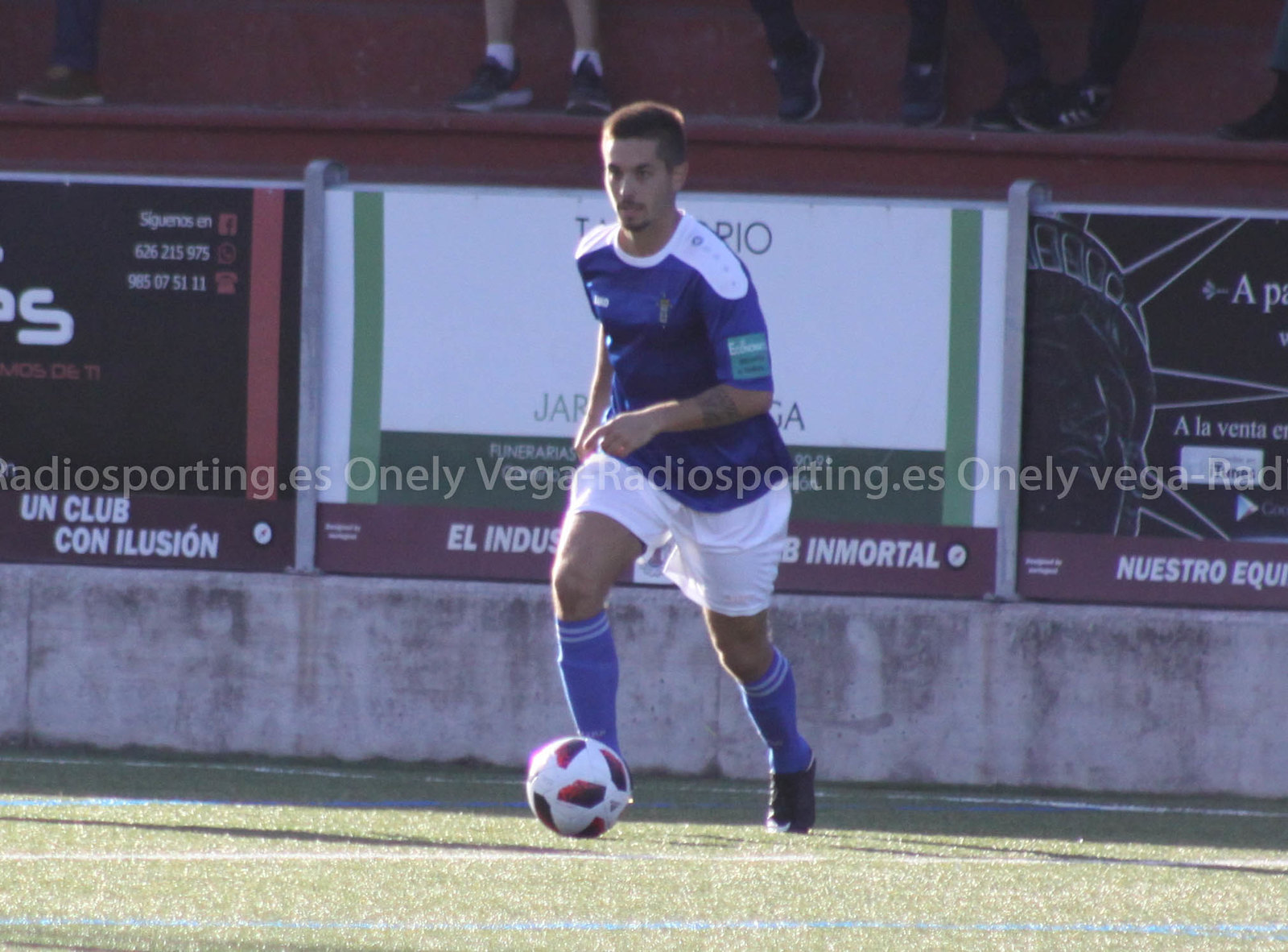A dynamic image captures a soccer player in action, clad in a blue and white kit. The player, who has short dark hair and a dark goatee, is seen dribbling a white soccer ball adorned with red and blue patches on a sunny day. His outfit consists of blue socks with white stripes at the top, white shorts, and a blue jersey with white shoulders. Notably, there is a green rectangle on the left sleeve of his jersey and he is wearing black shoes, likely with shin guards beneath his socks. The backdrop features a barrier wall lined with advertisements, written in Spanish, suggesting a Spanish-speaking location. In the stands behind, the feet of five fans are visible, accompanied by red seating. A repeated watermark, "O-N-E-L-Y, VegaRadioSporting.es," is prominently displayed across the center of the image. One of the sponsor logos on the far right side of the barrier includes an illustration resembling the Statue of Liberty, set against green-bordered signage.